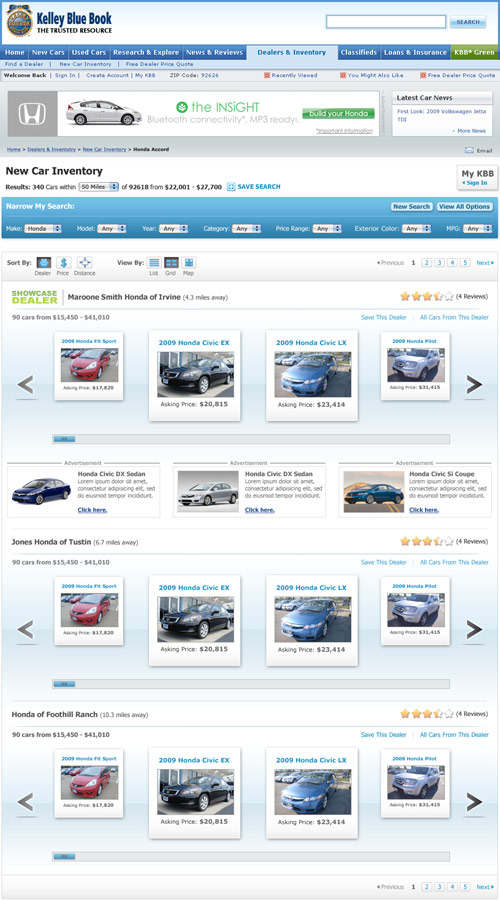The image showcases the homepage of the Kelley Blue Book website, widely regarded as a trusted automotive resource. Prominently displayed at the top is a navigation bar with various categories: Home, New Cars, Used Cars, Research and Explore, News and Reviews, Dealers and Inventory (highlighted as the active tab), Classifieds, Loans and Insurance, and KBB Green. 

A "Welcome Back" message invites users to sign in, create an account, or access their myKBB profile. The user's zip code is entered as 92424. There are sections for "Recently Viewed," "You Might Also Like," and an offer for "Free Dealer Price Quotes."

A featured Honda Insight, known for its Bluetooth connectivity and MP3 readiness, catches the eye under the "Build Your Honda" category. The screen also lists the latest car news and reviews, highlighting the 2009 Volkswagen Jetta.

Below, there is an extensive display of new car inventory spread across three rows, each featuring four cars. One notable dealership, Maroon Smith Honda in Irvine, located 4.3 miles away, lists 90 available cars ranging in price from $15,450 to $41,010, with an overall rating of 3.5 stars based on four reviews.